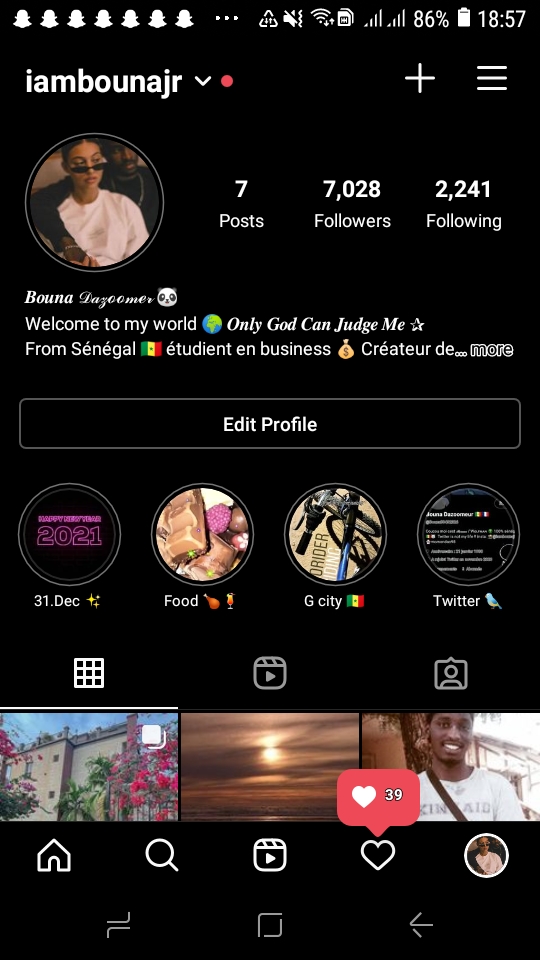This image is a screenshot taken from a cell phone displaying a social media app interface. 

In the top-right corner, there are various status icons including:
- The time "18:57"
- A battery symbol showing 86% charge
- Two full-bar wireless signals
- A SIM card icon
- A Wi-Fi signal symbol with up and down arrows
- A muted microphone icon
- A recycling symbol-like icon

In the top left, there are seven Snapchat icons. 

At the top of the social media interface is a username, "I am born a jar" with a dropdown menu icon next to it, accompanied by a red notification dot. On the opposite side in the top-right corner, there is a plus icon and a three-line menu icon indicating a dropdown menu.

The profile section just below this includes:
- A profile picture of a man in a black shirt with his arm around a woman in a white shirt
- An account with seven posts
- 7,028 followers
- The account is following 2,241 people

The description reads:
"Welcome to my world. Only God can judge me. From Senegal. Étudiant in business. Curator de..." followed by a "more" option to expand the text.

Below the description, there is an "Edit Profile" button and at the bottom of the screen are navigation icons including:
- A house (home)
- Magnifying glass (search)
- Video camera (video)
- Heart with 39 likes
- Profile picture (profile access)

The image captures both the detailed social media interface and the various phone status indicators.